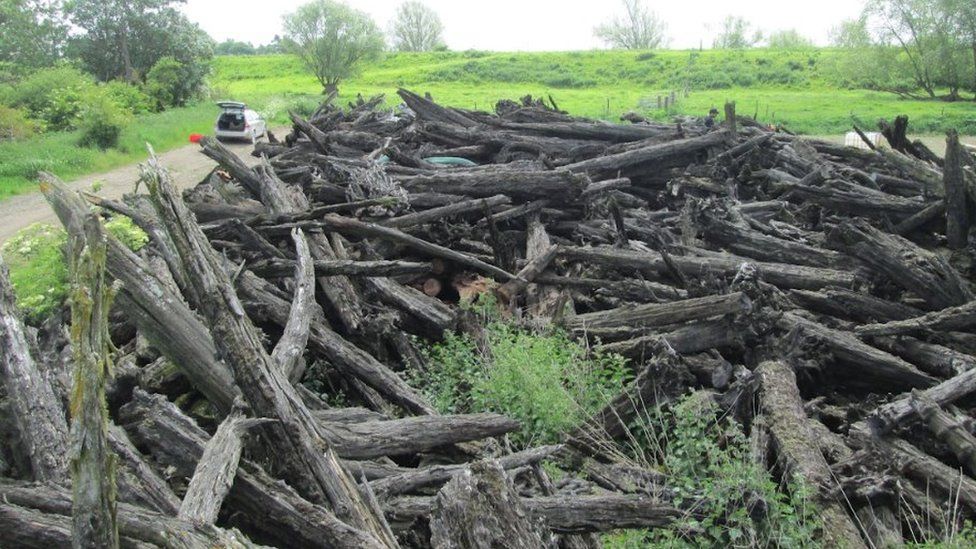This photograph features a very verdant, green landscape, dominated in the foreground by a large, weathered pile of cut logs, gray in color, which look as though they have been left out in the sun for a long time. This stack of aged wood resembles driftwood and includes fallen trees and cut-up tree stumps, mixed with some foliage growing through it. To the left, a dirt road extends diagonally into the distance, where a white van or station wagon is parked with its lift gate open. Nearby, an indistinct red patch is visible close to the vehicle. The background showcases a lush green field or marsh adorned with various types of trees, all under a cloudy sky. Additionally, a liquid tote can be seen to the right, just beyond the wooden pile, enhancing the sense of a remote, nature-filled setting.